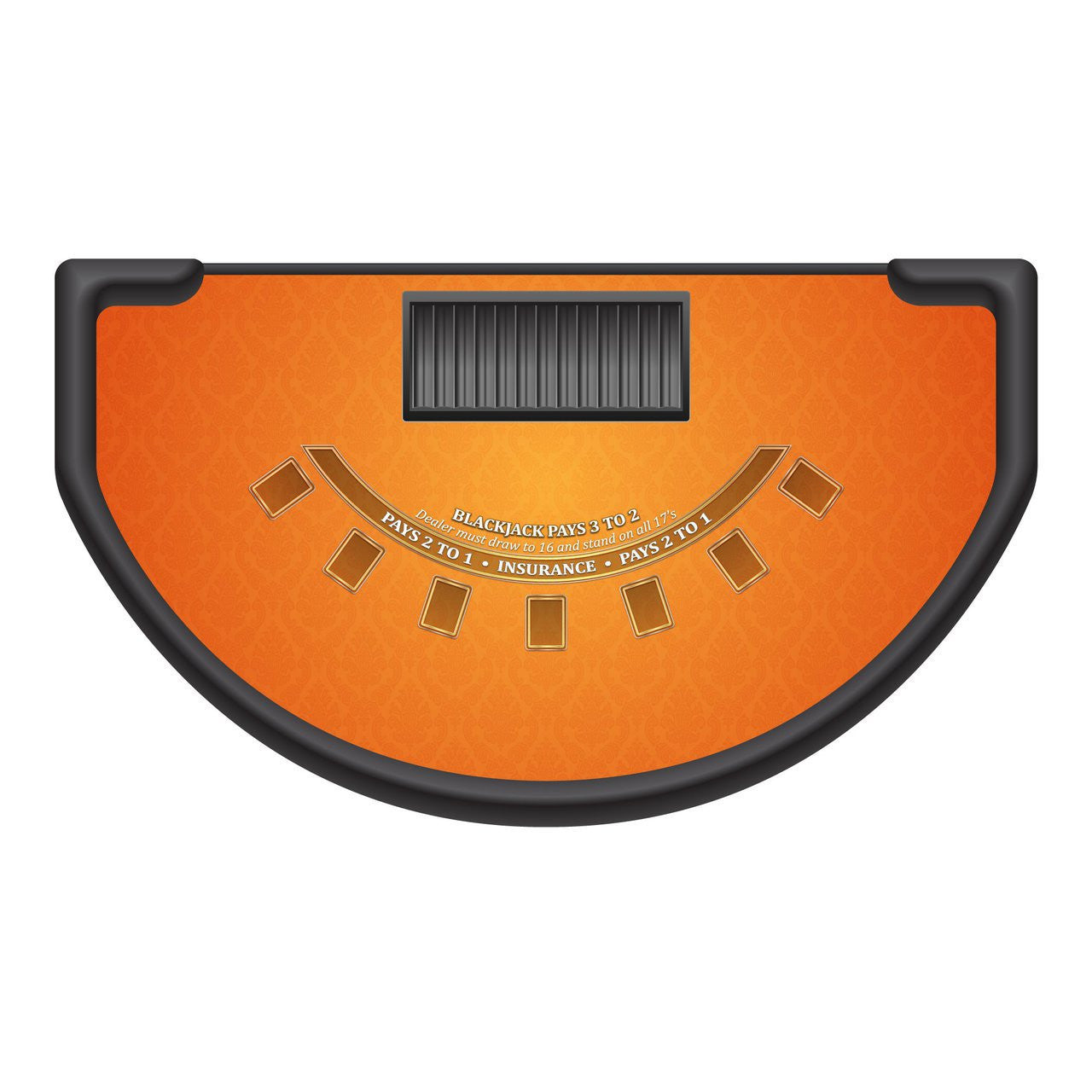The photograph is an overhead shot of a blackjack table, set against a white background. The table is shaped like a semicircle, with a black border and an orange playing surface. At the top center of the table, where the dealer would stand, there's a black rectangular slot, possibly for holding chips or money. The table features white text that reads, "BLACKJACK PAYS 3 TO 2," "DEALER MUST DRAW TO 16 AND STAND ON ALL 17s," "PAYS 2 TO 1," and "INSURANCE PAYS 2 TO 1." Along the curved edge of the table, there are outlined spaces for up to seven players to place their cards. The artwork includes representations of the card spaces in dark orange and gold, consistent with the overall orange theme of the table.